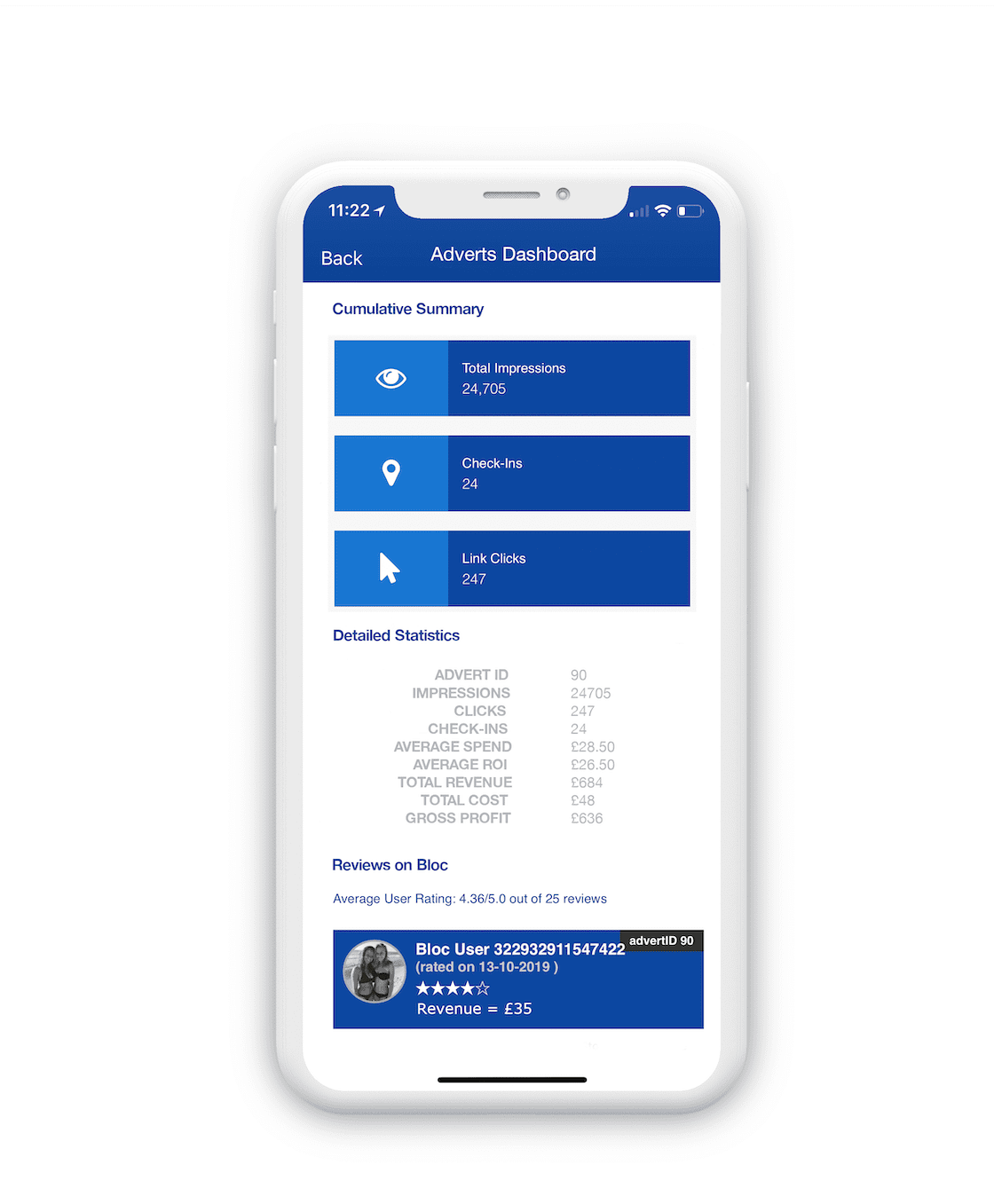The image displays the screen of a cell phone, presenting a comprehensive dashboard titled "Adverse Dashboards" at the top. The time displayed in the upper left corner is 11:22, along with standard symbols indicating Wi-Fi connectivity. The screen features a menu bar with options to navigate back, located at the top.

Beneath the title, the dashboard provides a cumulative summary of advertising statistics, which include:

- Total Impressions: 24,705.
- Check-ins: 24.
- Link Clicks: 247.

The top portion also includes various icons, such as an information icon indicating total impressions and a location pin symbol for check-ins.

Midway down the screen, there are detailed statistics separated into 9 categories. Though not all categories are labeled in the spoken description, they likely pertain to specific metrics or performance indicators. 

Additionally, there is information regarding reviews on "Block" (possibly a typo for 'Ploc' or another term), with an average user rating of 1.36 out of 5. 

At the bottom of the screen, there is another banner featuring an oval-shaped picture of two girls in bikinis, labeled "Block User." Another section provides an advertiser ID with the number "90" and a rating date of October 13, 2019, which received a rating of four stars. The revenue associated with this metric is marked as £35.

Overall, this detailed dashboard seems to offer a thorough analysis of advertisement performance metrics, reviews, and user ratings, presented in a visually structured manner.